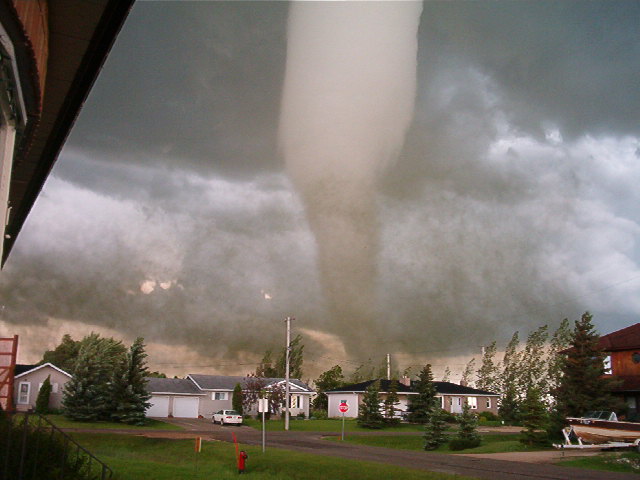The image depicts a massive tornado swirling ominously in the sky, threatening a small neighborhood. The funnel, narrower at the bottom and wider at the top, extends vertically to the top edge of the photo. A menacing purple sky frames the tornado, with darker shades concentrated on the top left and right corners. In the bottom third of the image, single-story homes with closed garage doors stand precariously, directly in front of the tornado. One of the houses on the far right features a dark red roof, with a boat on a trailer beside it. A white car is parked on a small street that runs in front of these homes. There's also a flagpole or streetlight near the houses and several trees visibly swaying to the right under the force of the winds. Prominently in the foreground, a red fire hydrant stands on a patch of grass, adding to the sense of foreboding as the storm closes in on the town.